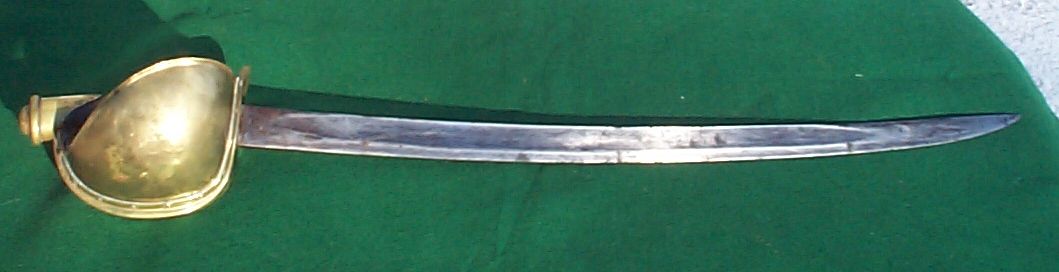This color photograph features a long, silver sword with a pointed tip, laying flat on a dark green velvet cloth. The sword's handle, situated on the left side, is gold and features a cup protector. The blade appears polished but shows signs of minor dents, indicating it has seen use. Despite these blemishes, the sword looks sharp and potentially usable. Shadows are visible in the upper left corner of the image, while the upper right corner displays a portion of a white surface, possibly a carpet. The photo, taken from a semi-above angle, showcases the entire length of the sword on the green cloth backdrop.